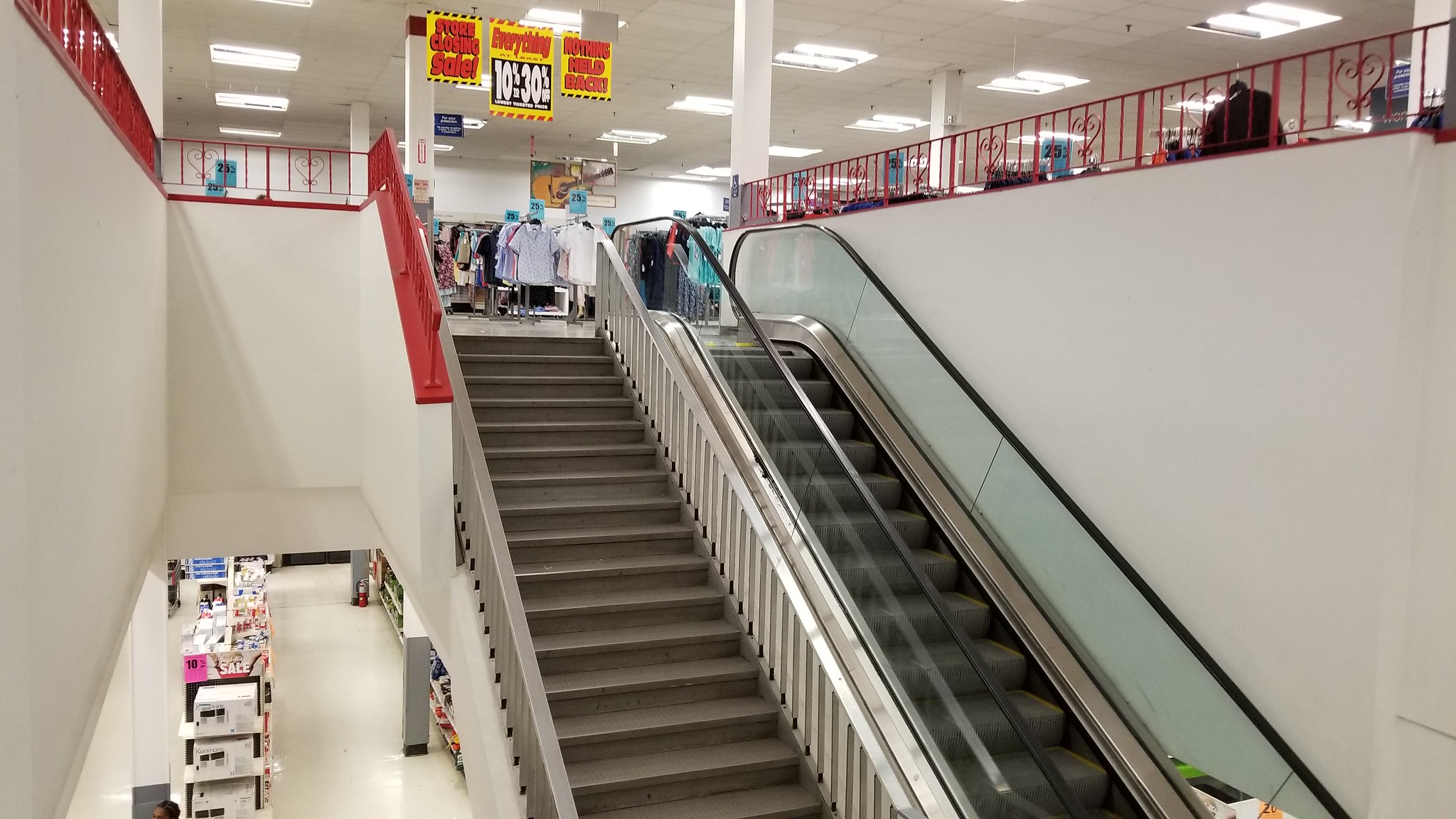This image captures a bustling department store interior featuring both an escalator and a staircase. The walls of the store are pristine white, enhancing the brightness provided by multiple rectangular lights affixed to the ceiling. The photograph reveals both the first and second floors of the store. On the upper floor, various clothing racks brimming with apparel are visible, alongside conspicuous yellow sale signs highlighting discounted prices. The escalator, positioned on the right, descends to the ground level, while a staircase on the left offers an alternative route between floors. A striking red iron railing stretches across the upper floor, adding a pop of color and serving as a safety barrier. On the ground level, several shelves and aisles can be observed, stocked with a variety of food items, indicating a diverse merchandise offering within the store.